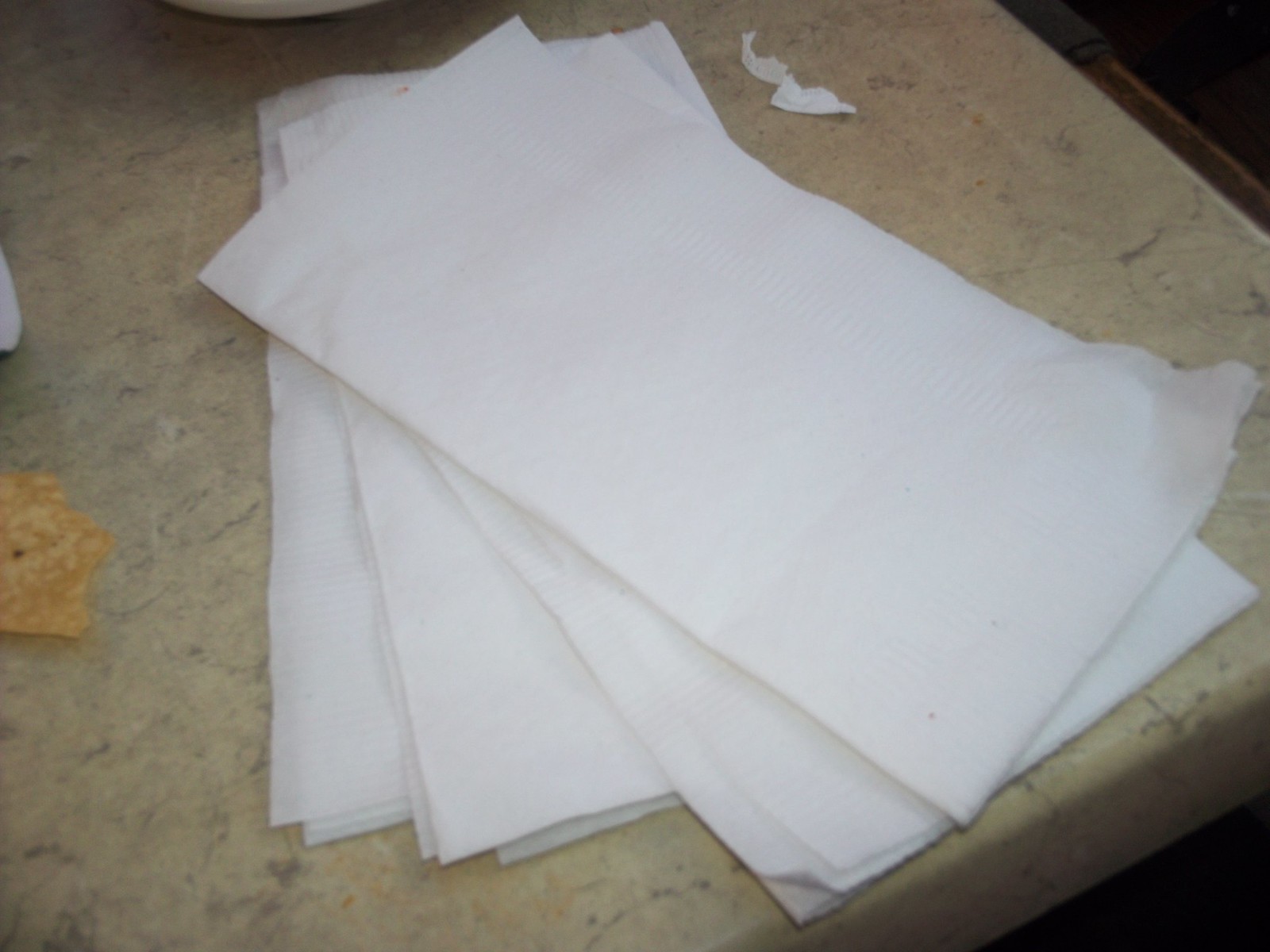This close-up photograph captures a light brown laminate or beige granite counter with subtle gray streaks. Prominently displayed are four white paper napkins, arranged in a fanned-out, slightly skewed stack. The napkin at the bottom lies almost horizontally to the camera, with each subsequent napkin tilted a bit more to the right, ending with the top one, which shows a slight wrinkle on its lower right-hand corner and a small red stain. A piece of torn white paper or a ripped-off end of a straw wrapper is also visible near the top. On the left side of the image, there is a solitary corn chip, light brown with much lighter tones of brown in the center, resting amongst the napkins. Surrounding these items, the edges of a white bowl and possibly other white objects peek into the frame.